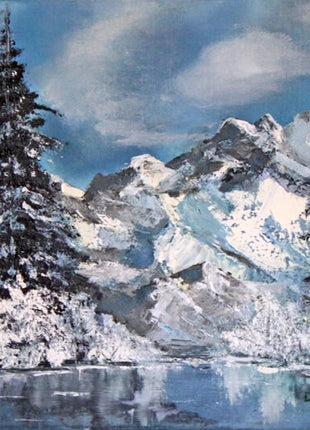This oil painting depicts a serene winter landscape dominated by a majestic, snowy mountain range. The tall conifer tree in the foreground, likely a pine or fir, stands on the left side, nearly reaching the height of the entire composition. The tree's base and middle sections are heavily laden with snow, causing some branches to droop under the weight, while the upper branches remain sparse. In the mid-ground lies a glassy, reflective body of water, possibly a frozen lake or river, mirroring the towering tree and portions of the snow-capped mountains. The mountain range itself, significant in both size and altitude, showcases a mix of dense snow coverage and patches of exposed rock. Above the mountains, the sky is partly cloudy, revealing streaks of blue amidst the white clouds. Notably, the painting contains no visible animals, humans, or writing, and the artist remains anonymous. The use of thick oil paints imparts a rich texture to the scene, particularly evident on the snow-laden hillside.